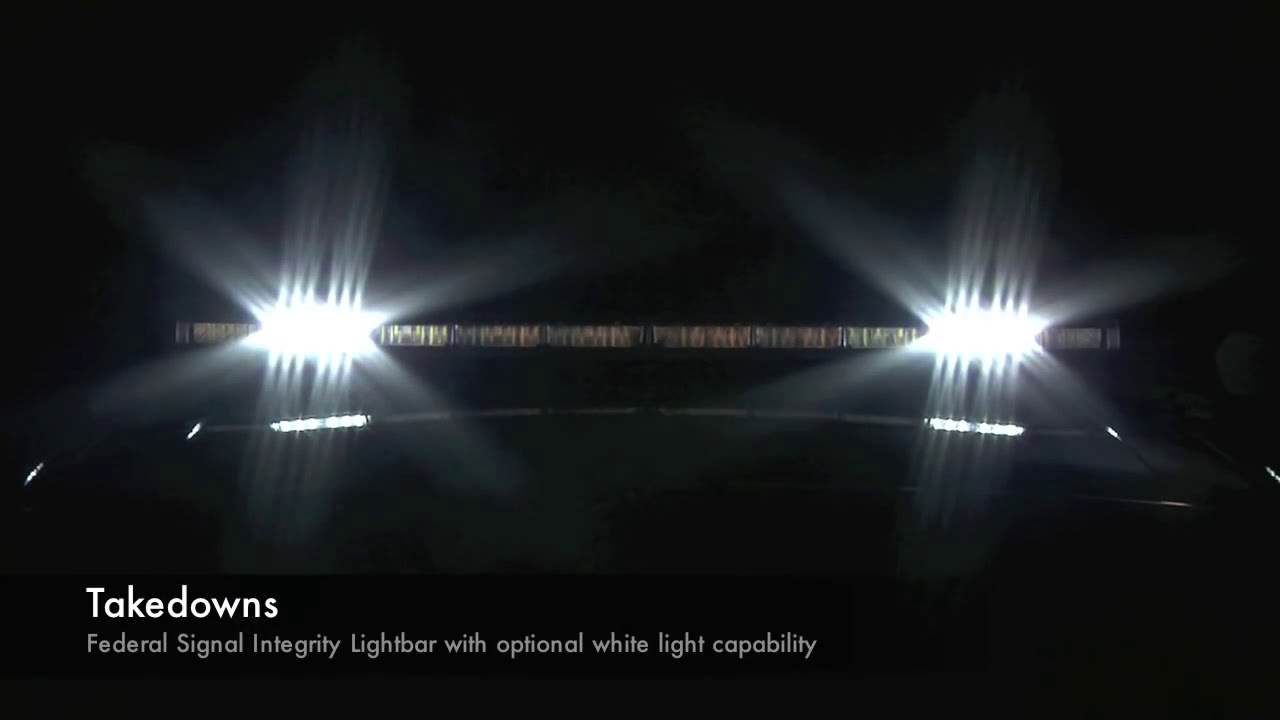The image depicts a mostly black and white, high-contrast photo of a light bar mounted on what appears to be a vehicle. The overall scene is very dark, possibly taken at night, with a near-total black background except for the illuminated light bar. This light bar features two brightly lit sections of lights, positioned towards the left and right ends, emitting a noticeable glare. 

Behind these lights is a thin, faintly yellow band stretching horizontally across the image, with another even thinner, slightly arced band beneath it. At the very bottom of the image, a black horizontal band displays white text. This text includes larger, bold letters spelling “Takedowns,” and below it, in smaller font, the text reads “Federal Signal Integrity Light Bar with Optional White Light Capability.”

Additionally, the curvature of the top part of a vehicle is subtly discernible beneath the bright lights, though it’s largely shadowed, integrating with the black backdrop. Despite the darkness, the entirety of the light bar across the top of the vehicle is visible, unlit sections bridging the illuminated extremes.